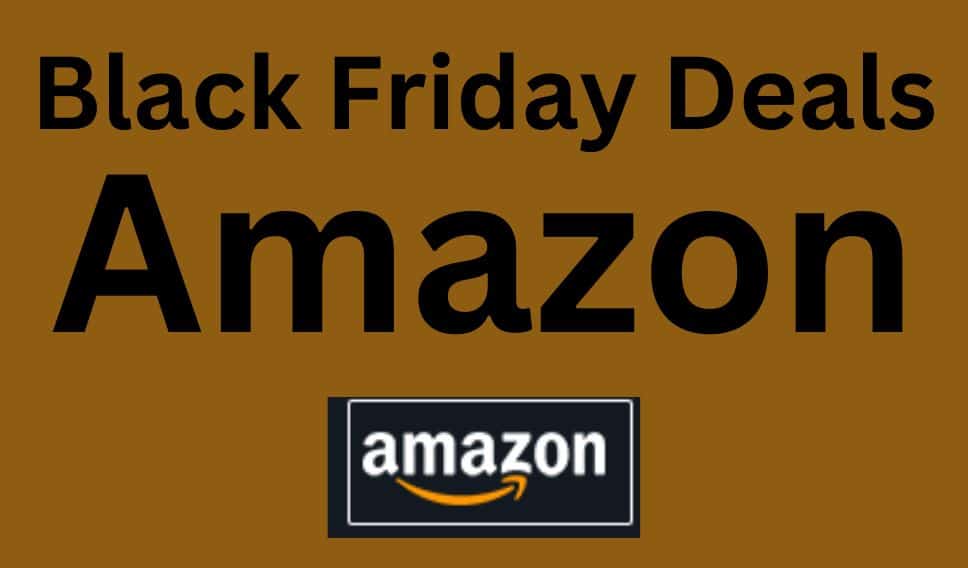The image features a large brown box prominently labeled with "Black Friday Deals" in bold black print. Below this text, there is a black rectangular box with a white outline. Inside this black box, the word "Amazon" is displayed in white letters. The iconic Amazon swoosh arrow, colored in vibrant orange, underscores the "Amazon" text. The combination of these elements clearly indicates that the box is part of Amazon's promotional materials for their Black Friday deals.